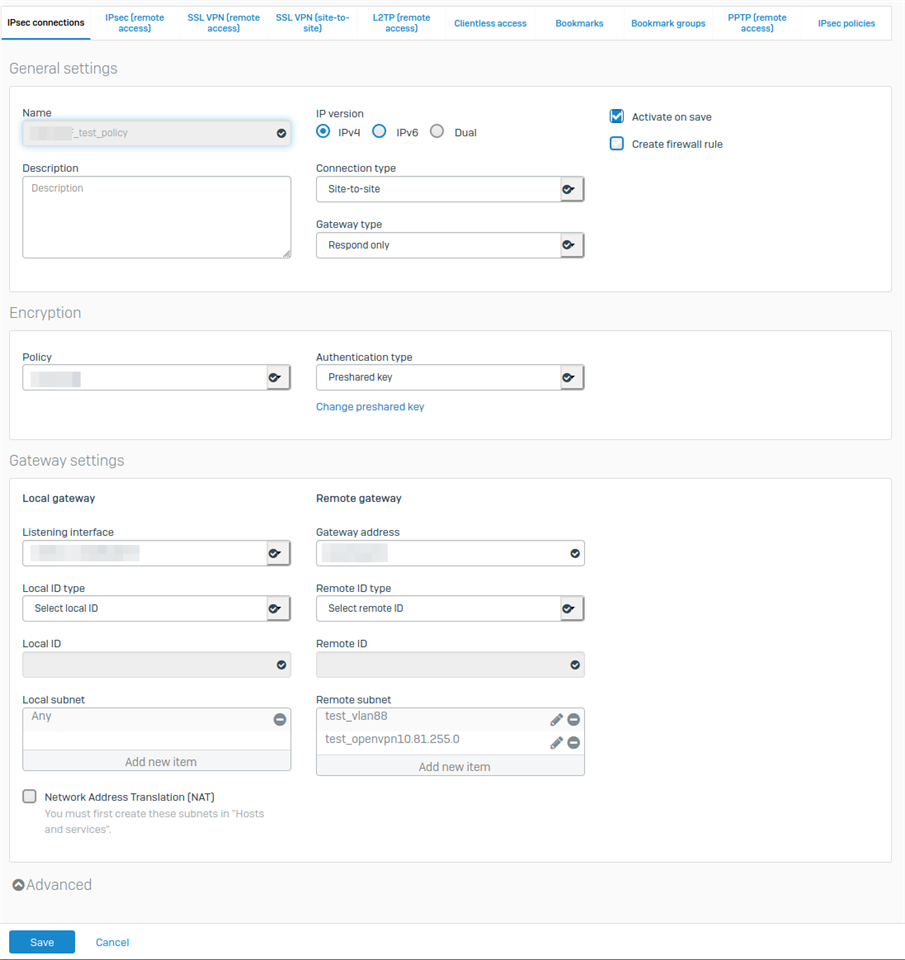The image displays a low-resolution screenshot of an application interface on a white background, with blue as the primary accent color throughout. 

At the top, there is a barely legible horizontal list of ten tabs, each represented by blue text. The tab on the far left is highlighted with black text and a blue underline, indicating it is currently selected. Below the tab list, the heading "General Settings" is visible.

The interface includes various interactive elements, starting with two text entry boxes labeled "Description" and "Name." Below these, there are three radio buttons lined horizontally, with the leftmost one selected. Further down, there are two drop-down menus with text that is unreadable in this image. A selected checkbox depicted in blue, and an unselected checkbox beneath it, appear next.

Towards the bottom of the interface, there is an arrangement of drop-down menus: five on the left side and five on the right side. Finally, at the very bottom, there are "Save" and "Cancel" options; the "Save" button is blue with white text, and the "Cancel" option is rendered in blue text without a button but remains interactive.